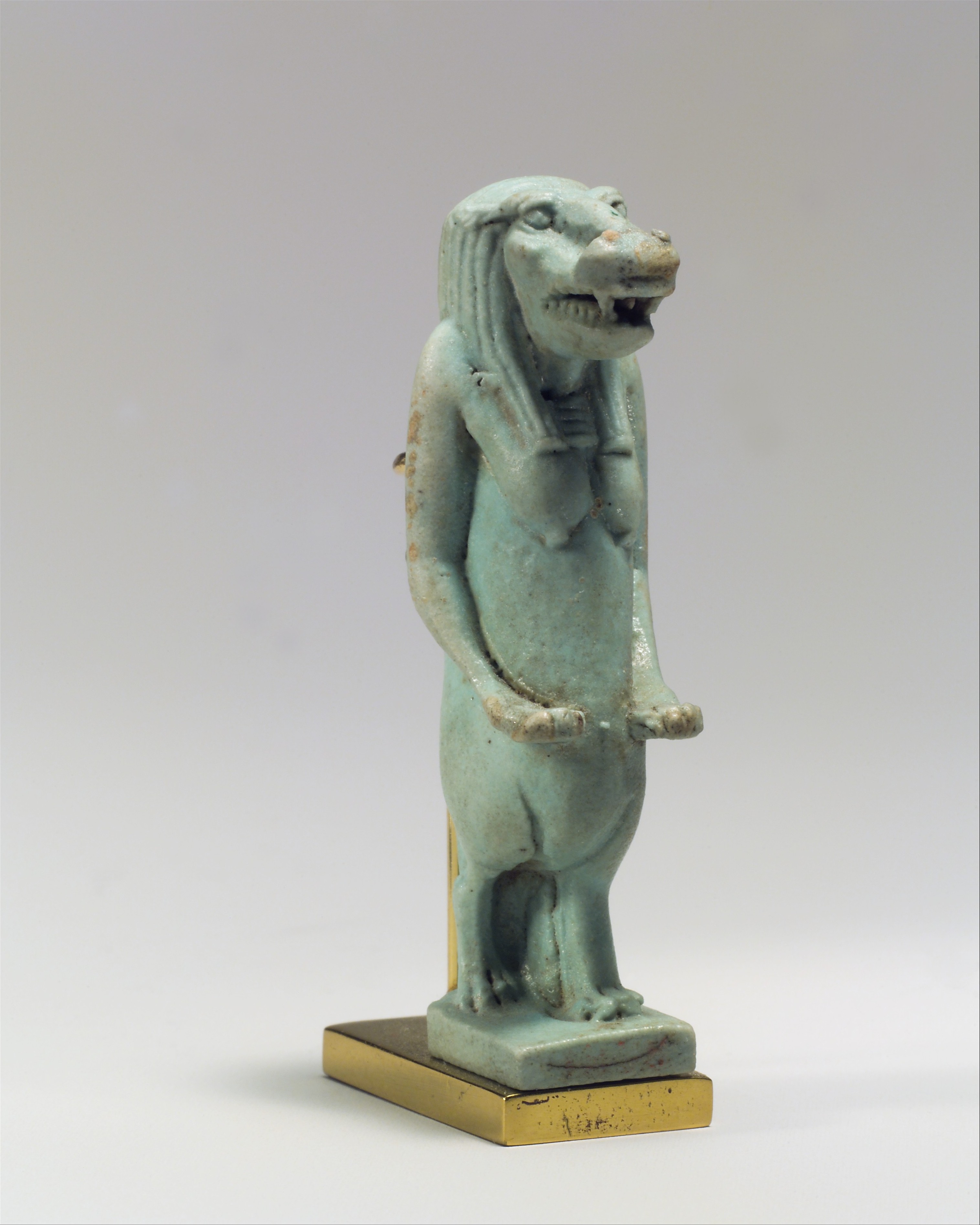The image features a detailed jade statue set against a plain gray background, likely intended for museum display or educational text. The statue exhibits the figure of a dog-like creature standing erect on two short back legs. It has a long snout with prominent canine teeth and a slightly open mouth, showcasing two sharp fangs. The creature’s eyes and eyebrows are discernible on its flat head, and it has a notably large nose. Covering its head and extending down to its shoulders is long, dreadlock-like hair. Additionally, it features sagging, pancake-shaped breasts with prominent nipples and an intricate necklace around its neck. The creature's elongated arms hang down in front, ending in dog-like paws. The statue’s base is square and rests atop a gold-colored block, with an additional support stand behind it.